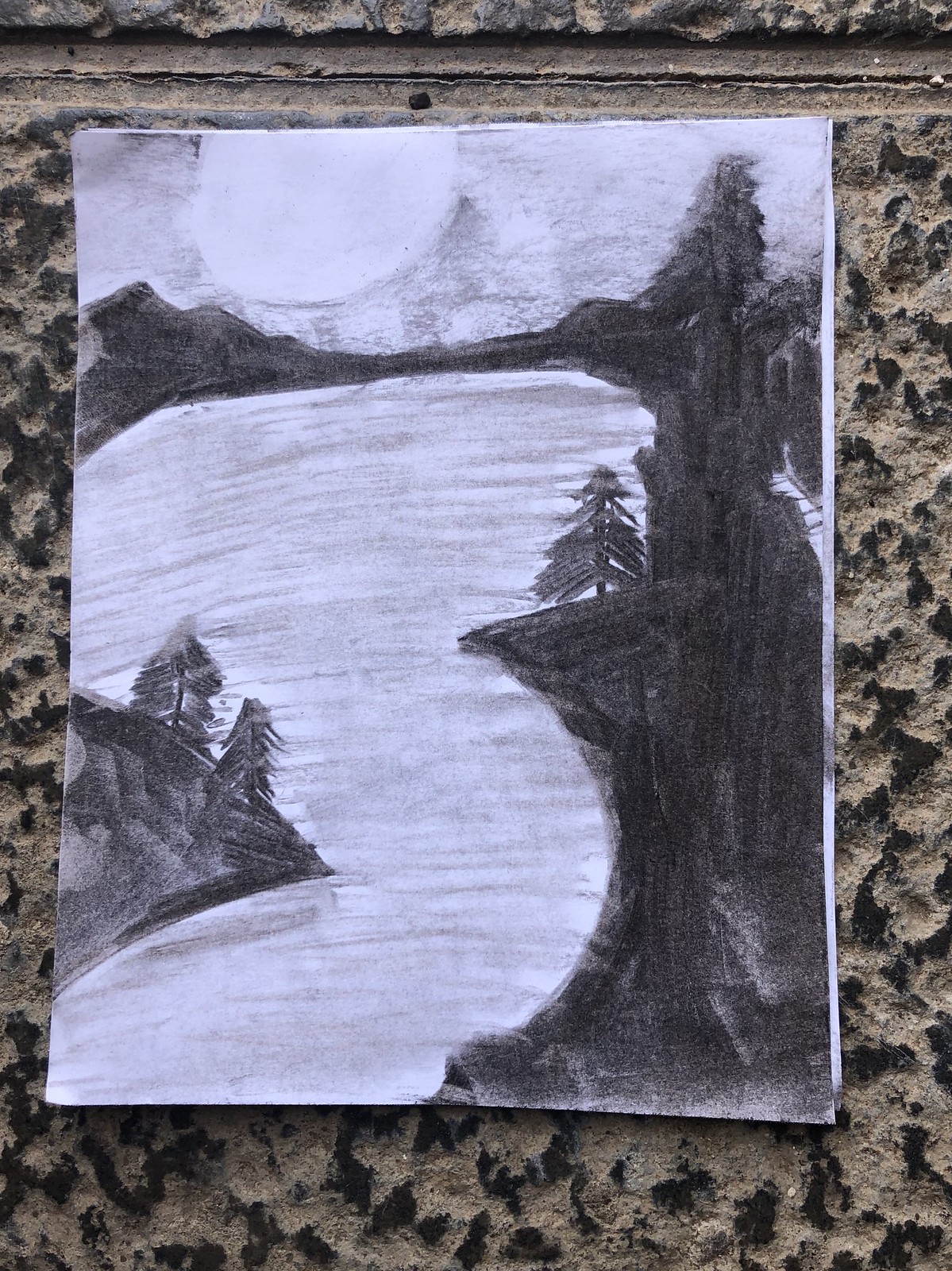This image features a meticulously detailed black and white drawing, created on standard printer paper. The artwork showcases various types of trees, representing a natural environment. The composition includes a towering mountain-like formation, adding a sense of grandeur to the scene. The trees and other elements are rendered in dark tones, contrasting sharply against the white paper. The background suggests a rocky or stony setting, possibly an outdoor surface or a stone table, illuminated by ample daylight. The intricate details and vivid contrast of the black ink on white paper indicate that the artist invested considerable time and effort into this well-executed piece.